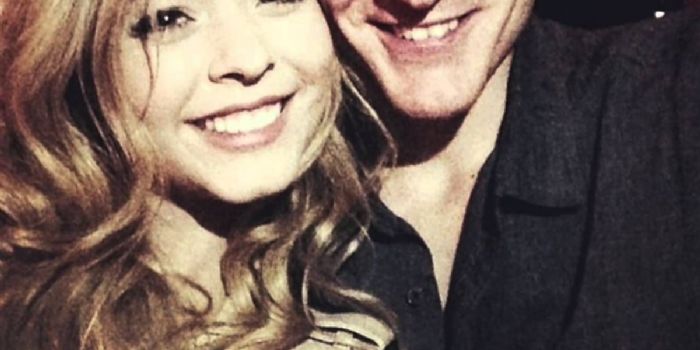In the close-up, cropped image, a happy couple is seen taking a selfie. The man's face is cut off at the nose, revealing his smile and a glimpse of his chest through an open black dress shirt. The woman's face is partially visible, with her right eye cropped out. She has wavy, dirty blonde hair, brown eyes, and is sporting a bright, vibrant smile with just her top teeth showing. She's likely wearing a black coat, though it's partially obscured by the cropping. Both appear to be of European and Caucasian descent. The picture, seemingly taken at night with flash, has an intimate and cheerful ambiance.